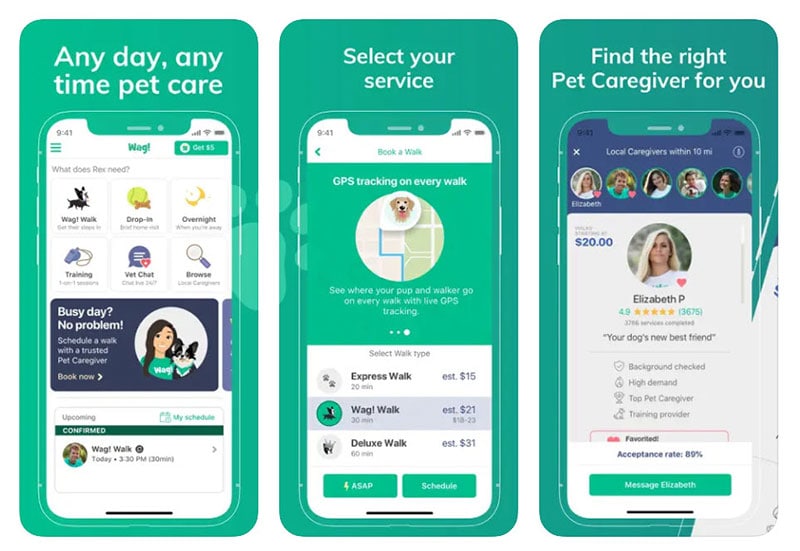### Detailed Descriptive Caption:

The image showcases a mobile app with three different screens, each displayed on a green-backgrounded phone. 

- **First Phone (Leftmost Screen):**
  1. The phrase "Any day, anytime pet care" is prominently displayed along with the number "941".
  2. Below this, the app has several navigation buttons: a green button labeled "Got it" and another reading "What does Rex need?".
  3. Six options are presented in boxed icons: "Wag Walk," "Drop-in," "Overnight," "Training," "Vet Chat," and "Browse".
  4. A large blue box with the heading "Busy day? No problem." features a circular image of a girl with a dog.
  5. The box also includes the text: "Schedule a week with a trusted pet caregiver. Book now".
  6. At the bottom, there's another box titled "Upcoming" which shows "My Schedule" with a green label reading "Confirmed" underneath "Wag Walk", accompanied by an illustrative image.

- **Second Phone (Middle Screen):**
  1. The heading "Select Your Service" leads into the option "Book a Walk".
  2. There is a left-pointing arrow and the phrase "Green GPS tracking on every walk", accompanied by an icon of a map with a dog’s picture.
  3. Navigation dots at the bottom highlight that this is the third screen in a sequence.
  4. A white box titled "Select Walk Type" presents options:
     - "Express Walk" for $15
     - "Wag Walk" for $21 (highlighted in blue)
     - "Deluxe Walk" for $31
  5. Two green buttons labeled "ASAP" and "Schedule Me" are available for immediate or planned bookings.

- **Third Phone (Rightmost Screen):**
  1. The title "Find the Right Pet Caregiver" is displayed prominently.
  2. A blue box with an X in the corner describes "Local caregivers within 10 miles" and shows images of five different people.
  3. A large blue box beneath features a circular image of a young woman titled "Elizabeth P". 
  4. Details include her rate of $20, an acceptance rate of 89%, and a button labeled "Message Elizabeth" in green.

Each screen visually guides the user through the process of scheduling a service, selecting a walk type, and finding a caregiver, ensuring a comprehensive and user-friendly experience.